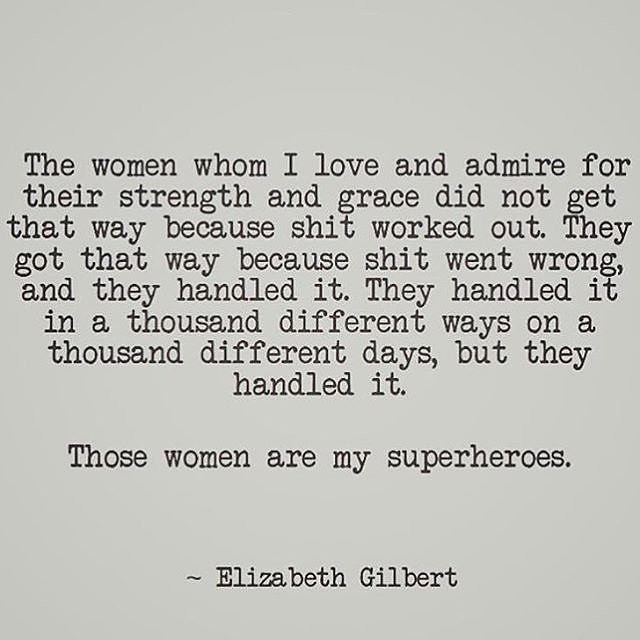The image is a large square with a solid gray background, featuring centered text in a black typewriter font. The text reads, "The women whom I love and admire for their strength and grace did not get that way because shit worked out. They got that way because shit went wrong and they handled it. They handled it in a thousand different ways on a thousand different days but they handled it." Following a space, it continues, "Those women are my superheroes." At the very bottom, it is signed with an approximate symbol and "Elizabeth Gilbert." The quote is positioned slightly lower in the frame, with about a quarter of the space left blank at the top.